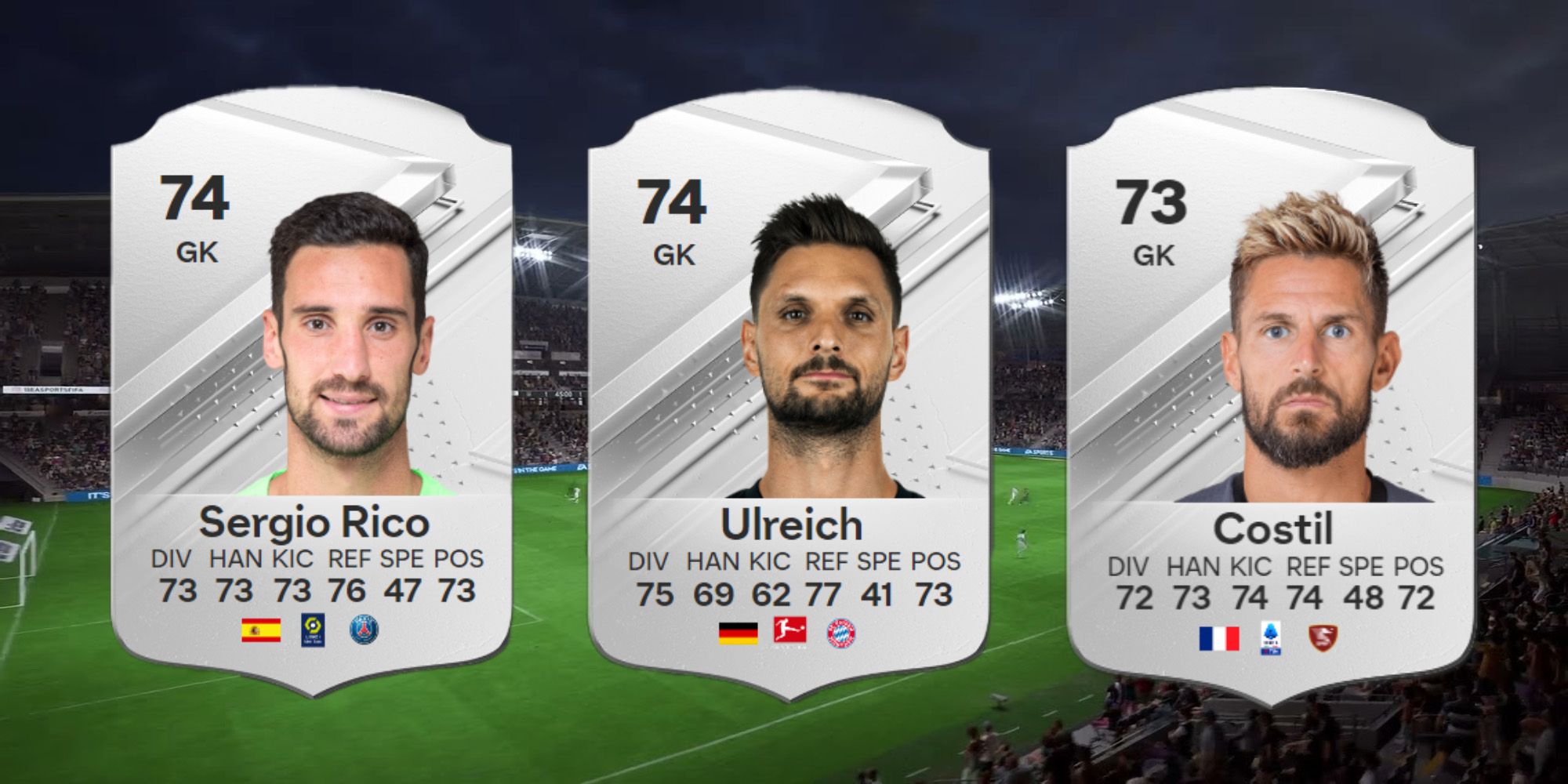The image is a detailed screenshot from a TV or web broadcast of a nighttime soccer match, showing a packed stadium. The night scene is brightly illuminated by stadium lights. Dominating the image are three shield-shaped overlays positioned side-by-side in the center, each featuring a different soccer player and detailed statistics. Each shield contains a high-quality photograph of a player and is bordered by a silver and gray design. The left shield shows Sergio Rico, a male with short dark hair and beard, labeled with "74 GK" in black text at the top, followed by his name and additional stats. The center shield features Ulrich, a dark-skinned male with short black hair and a beard, also marked with "74 GK" and his name beneath. The right shield highlights Costil, whose hair has bleached highlights and who has a dark beard, noted with "73 GK" at the top and his name and stats below. The background field and fully occupied bleachers add context to the setting, emphasizing the real-time broadcast nature of the image.